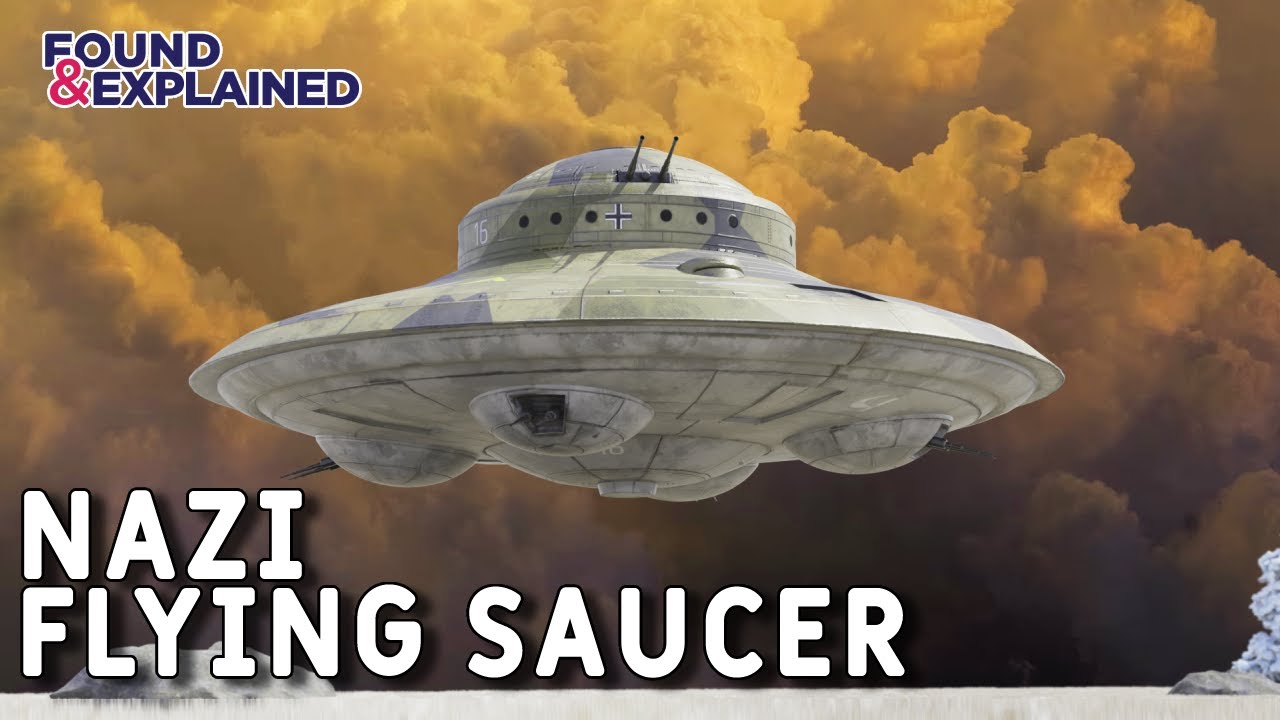The image features a gray camouflage-patterned flying saucer prominently displayed against a dramatic sky filled with turbulent clouds. The saucer is detailed with several bulges underneath that appear to be gun turrets pointed in various directions, as well as two prominent cannons extending towards the top right. At the very top left corner of the image, the text "Found and Explained" is written in a dark purple color with a white outline. Dominating the bottom left, in large, bold, capitalized white letters with a black outline, is the phrase "NAZI FLYING SAUCER." The background showcases a sky filled with clouds that transition from a lighter orange at the top to a darker orange or black towards the bottom, contributing to a stormy, ominous atmosphere. On the bottom right, two gray rocks are visible.